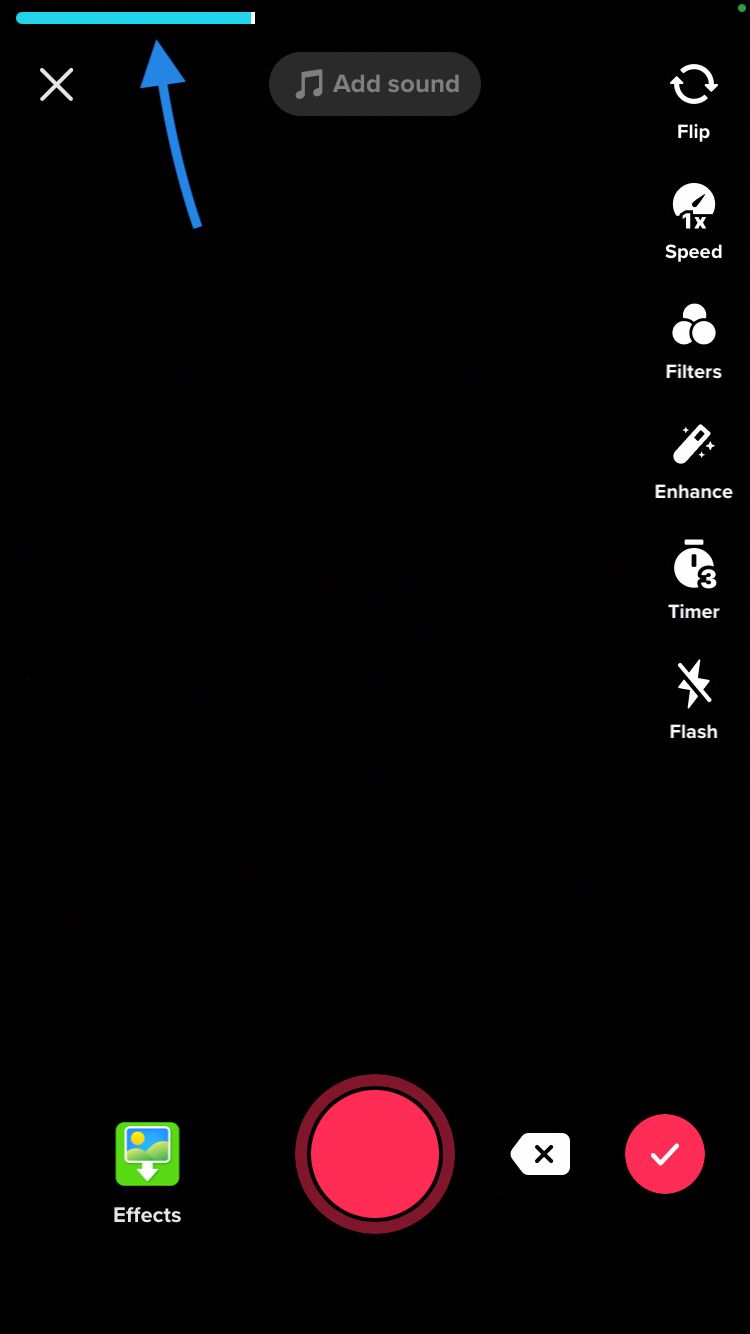Screenshot of the TikTok app showcasing the video creation interface: 

The image depicts the video recording section of someone's TikTok page with a solid black background. On the right side of the screen, there's a vertical toolbar featuring several video adjustment options: a camera flip icon, a speed adjustment icon labeled "1x," three circles for filters, a sparkling pen for enhancement, a clock for the timer, and a crossed-out lightning bolt for flash settings.

At the bottom of the screen, the left corner displays an effects icon, characterized by a green square with a sun image. In the center, there's a prominent red record button encircled by a light red border. Moving to the right, we find an "X" button for canceling actions and a red checkmark for confirming recordings.

At the top portion of the screen, on the left side, there's an "X" icon to exit the video creation page. Centrally located is a long cylindrical button with a music note icon and the label "Add Sound." At the very top of the interface, a blue progress bar indicates the duration of the current video, accompanied by a darker blue arrow pointing at the progress bar to highlight the video's elapsed time.